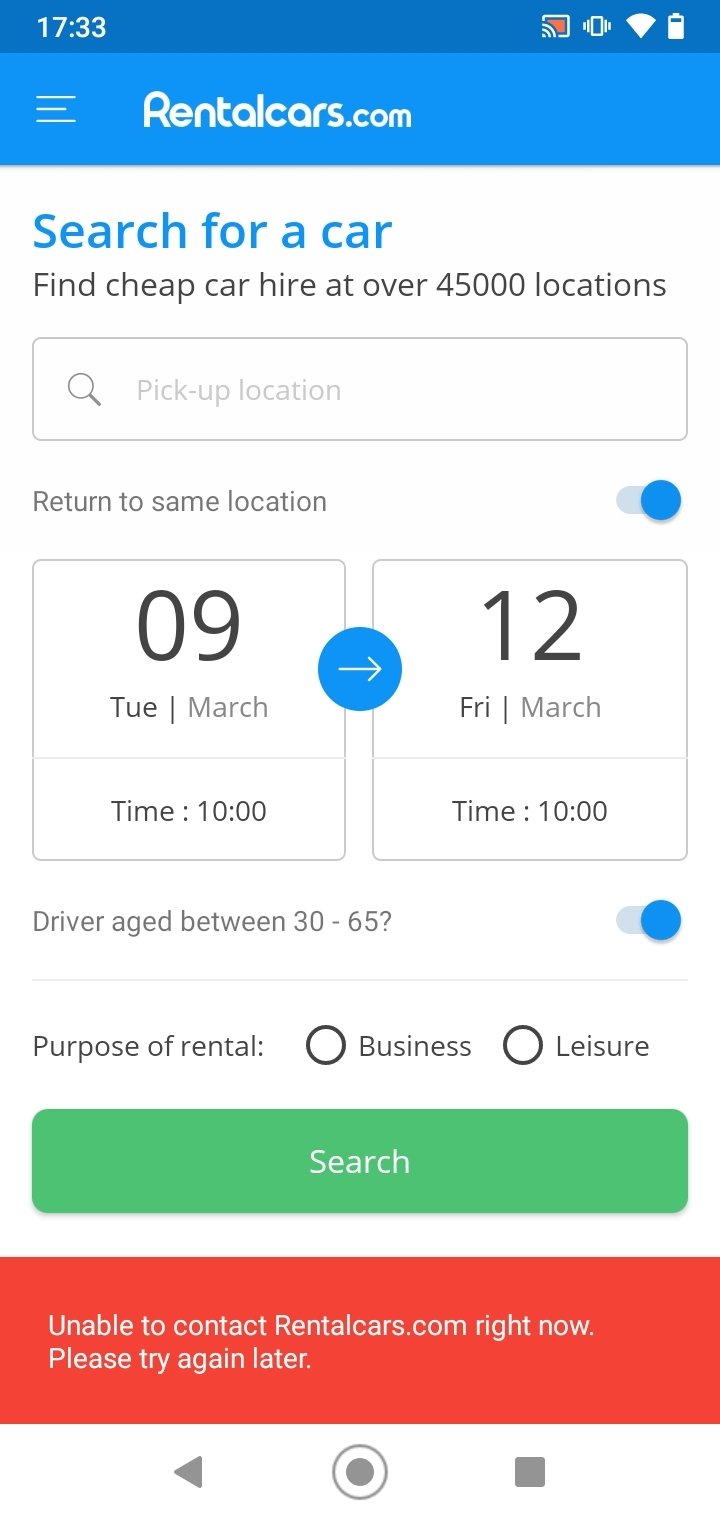The image is a detailed screenshot of the rentalcars.com webpage viewed on a phone. At the top, the website's name, "rentalcars.com," is clearly visible, indicating the source. The page features a string of informational text starting with "Search for a car," followed by a tagline "Find cheap car hire at over 45,000 locations." 

Central to the page is a prominent search bar placeholder labeled "Pick up location," designed for users to input their desired rental car location. Just below this, there is a toggle switch marked "Return to same location," which users can enable or disable based on their preference.

The most substantial portion of the screen showcases the date and time selection for the car rental. The specified rental period stretches from Tuesday, March 9th, to Friday, March 12th, totaling a three-day span, with both pick-up and drop-off times set at 10 a.m. 

Underneath the date and time fields, there is another toggle switch option labeled "Driver age between 30 to 65," allowing users to specify if the driver's age falls within this range. 

Following this is a section labeled "Purpose of rental," where users can select between two options: "Business" or "Leisure." At the bottom of the screen, a conspicuous green "Search" button is displayed, enabling users to finalize their input and initiate the search for available rental cars based on the provided criteria.